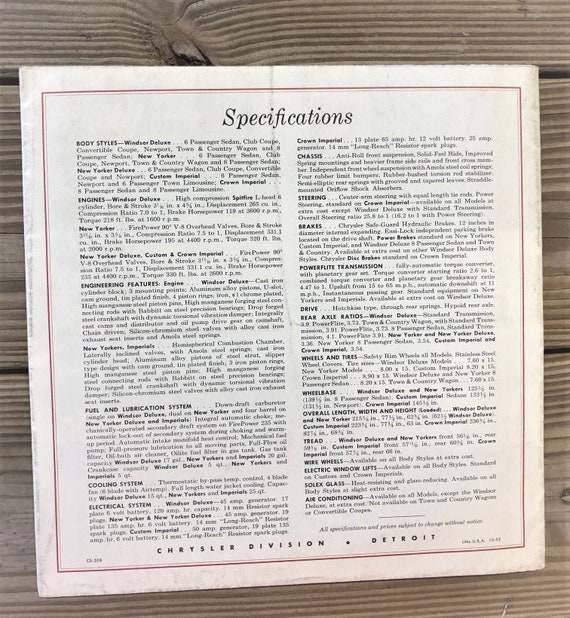The image displays a detailed specifications page, bordered in red, with a black italicized heading that reads "Specifications." The page thoroughly outlines various aspects of a car, including body styles, engines, engineering features, fuel and emission systems, powerful transmission, drive, as well as wheels and tires. Each category is presented with bold headings followed by descriptive text. Notably, the specifications mention various body styles such as "window deluxe" and "New Yorker Deluxe," and include the information "Chrysler Division, Detroit" at the bottom of the page.